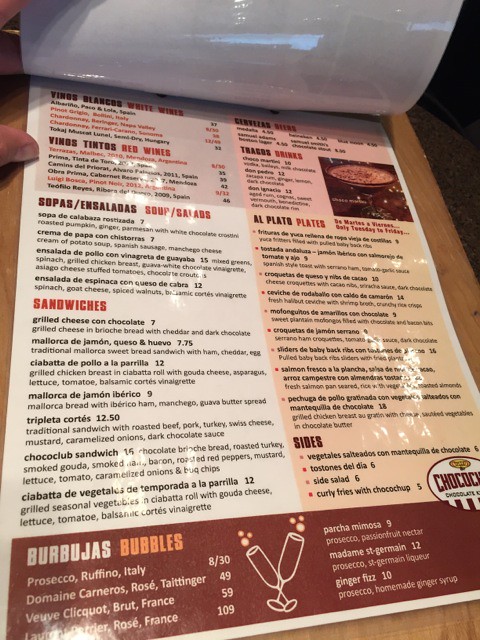Detailed Caption for the Photographic Image of a Menu:

A detailed photograph captures a pristine menu placed on a clipboard, showcasing its predominantly white design with tasteful shades of red throughout. The menu appears to be in the process of being opened to the second page, which boasts a high-gloss lamination, giving it a sleek and polished look. Light reflections are visible on the laminated surface, adding a subtle gleam to the white backdrop of the first page. 

At the top section of the menu, bold headings categorize the offerings: "Beings," "Tintos (Red Wines)," "White Wines," "Sopas y Saladas (Soups and Salads)," "Sandwiches," "Beers (Cervezas)," "Drinks," "Plates," and "Sides." Each category is thoughtfully sectioned, guiding patrons through their culinary options.

At the bottom of the menu, a long, prominent red banner highlights an assortment of bubbly delights. This banner lists several options such as "Bubbles," "Prosecco Rufino from Italy," "Domain Carneros Rosé," and "Taittinger." Additionally, it details two types of Champagne: "Brut from France" and "Rosé from France." The selection is rounded off with refreshing mimosas and an enticing "Ginger-Fizz" made with Prosecco and homemade ginger syrup. This detailed, glossy menu promises a diverse and delectable dining experience.